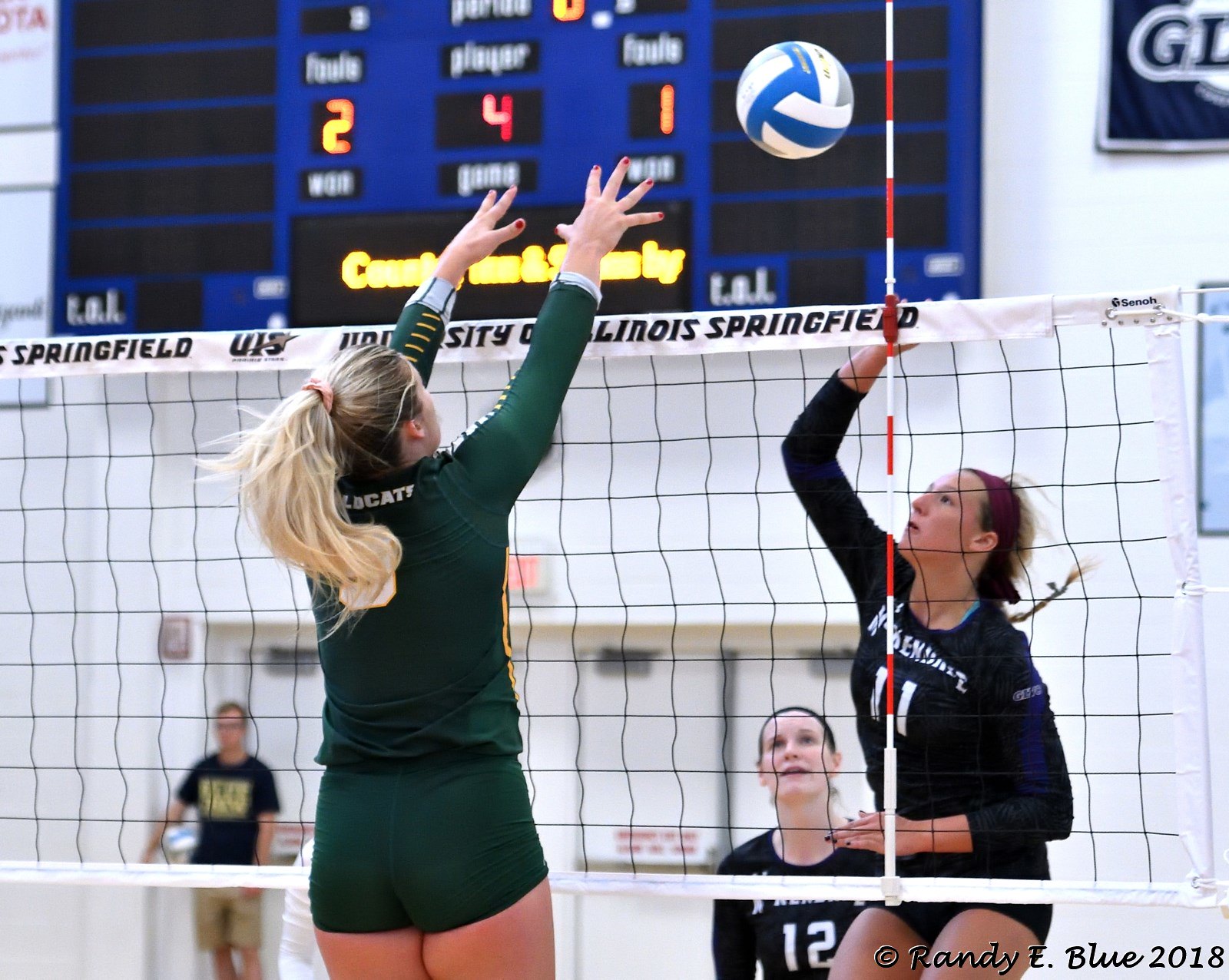This detailed photograph captures a high-energy moment in a women’s volleyball game. The image, oriented horizontally, features action on both sides of the net, which is held up by blue posts. The net has the inscription "University of Illinois Springfield" across the top. At the center of the action, a woman in a green long-sleeved uniform and shorts is leaping with both hands raised, ready to block or deflect a spike from her opponent. On the opposite side, a player in a blue uniform, presumably having just hit the white volleyball with blue stripes, is airborne as well. Supporting the blue-uniformed player is another team member wearing the number 12, who is attentively watching the ball’s trajectory. 

The scene is set in an indoor gymnasium, with a prominent blue scoreboard mounted on the white wall above the players. The scoreboard shows one team with a score of 4 and the other with a score of 2, along with an additional unreadable number 1. In the background, a male spectator stands near the exit doors, observing the unfolding match. The photograph is credited to Randy E. Blue, 2018, as noted by a copyright in the bottom right corner. The players' hair is neatly tied back, ensuring it doesn't interfere with their performance.